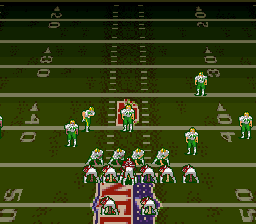A pixelated screenshot from a classic football video game captures a moment on the gridiron. Despite its retro graphics, the image vividly depicts the action. The detailed pixels reveal the NFL logo at the center of the field. Two teams are clearly distinguishable: one clad in red uniforms with white pants, the other in white uniforms with green pants and green lettering. The yard markers—50, 40, 30, and 20—are visible, segmenting the field. On the green team's side, partially obscured by a player, a red logo peeks through. Dashed lines traverse the field, guiding the eye towards the yard markers. The square image seems small, and the lighting darkens towards the top, casting a subtle shadow over the scene. Directional arrows are visible, pointing towards the 40 and 30-yard lines, adding to the strategic essence of the moment captured.